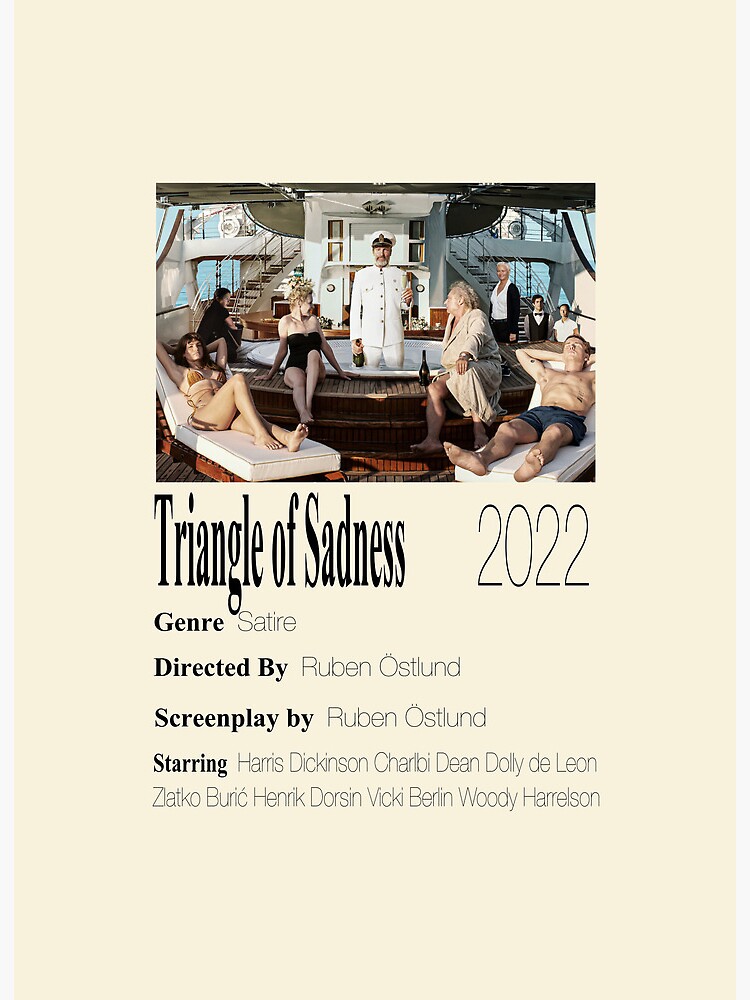The image is a portrait-layout brochure with a cream or peach background. At the top, there is a rectangular photograph depicting a luxurious scene on a yacht. In the photograph's center, a boat captain dressed in an all-white uniform and hat stands in a white hot tub with wooden deck borders. Surrounding the captain are two women and two men in bathing suits. On either side, a young woman and a man lounge on white cushioned chairs, while an older couple sits on the jacuzzi's edge, with a bottle of wine nearby. The captain also appears to be holding a bottle. Below the photograph, in bold black text, the brochure reads: "Triangle of Sadness (2022), Genre: Satire, Directed by Ruben Östlund, Screenplay by Ruben Östlund, Starring Harris Dickinson, Charlbi Dean, Dolly De Leon, Zlatko Burić, Henrik Dorsin, Vicki Berlin, Woody Harrelson."